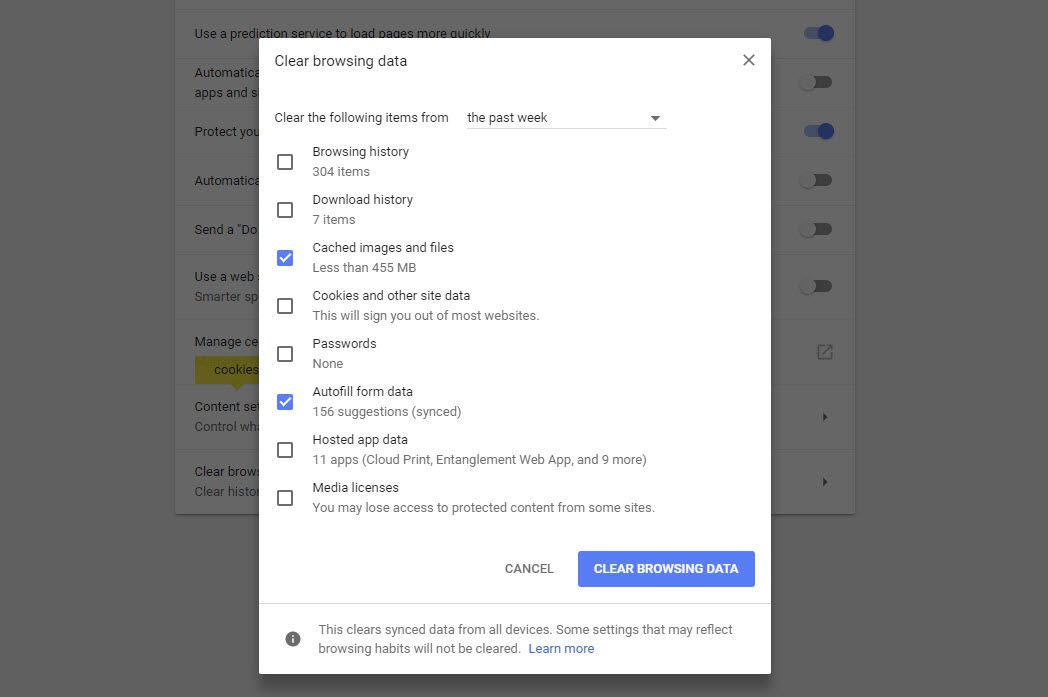This is a detailed screenshot of the "Clear browsing data" settings page in Google Chrome. The user has selected to clear data from "the past week." The selectable items for clearing browsing data are listed with their statuses:

1. **Browsing history (304 items)** - Not checked.
2. **Download history (7 items)** - Not checked.
3. **Cached images and files (less than 455 MB)** - Checked.
4. **Cookies and other site data** - Not checked, with a note saying that this will sign you out of most websites.
5. **Passwords** - Not checked.
6. **Autofill form data (156 suggestions synced)** - Checked.
7. **Hosted app data (11 apps, including Cloud Print and Entanglement Web App)** - Not checked.
8. **Media licenses** - Not checked, with a note indicating that you may lose access to protected content from some sites.

At the bottom of the window, there are two actionable buttons:
- **CLEAR BROWSING DATA** (white text on a blue button).
- **CANCEL**.

In the background, a partially visible grayed-out window contains additional settings with toggle switches, although the specific details are obscured by the forefront window.

At the very bottom, there is fine print information:
"This clears synced data from all devices. Some settings that may reflect browsing habits will not be cleared. Learn more."